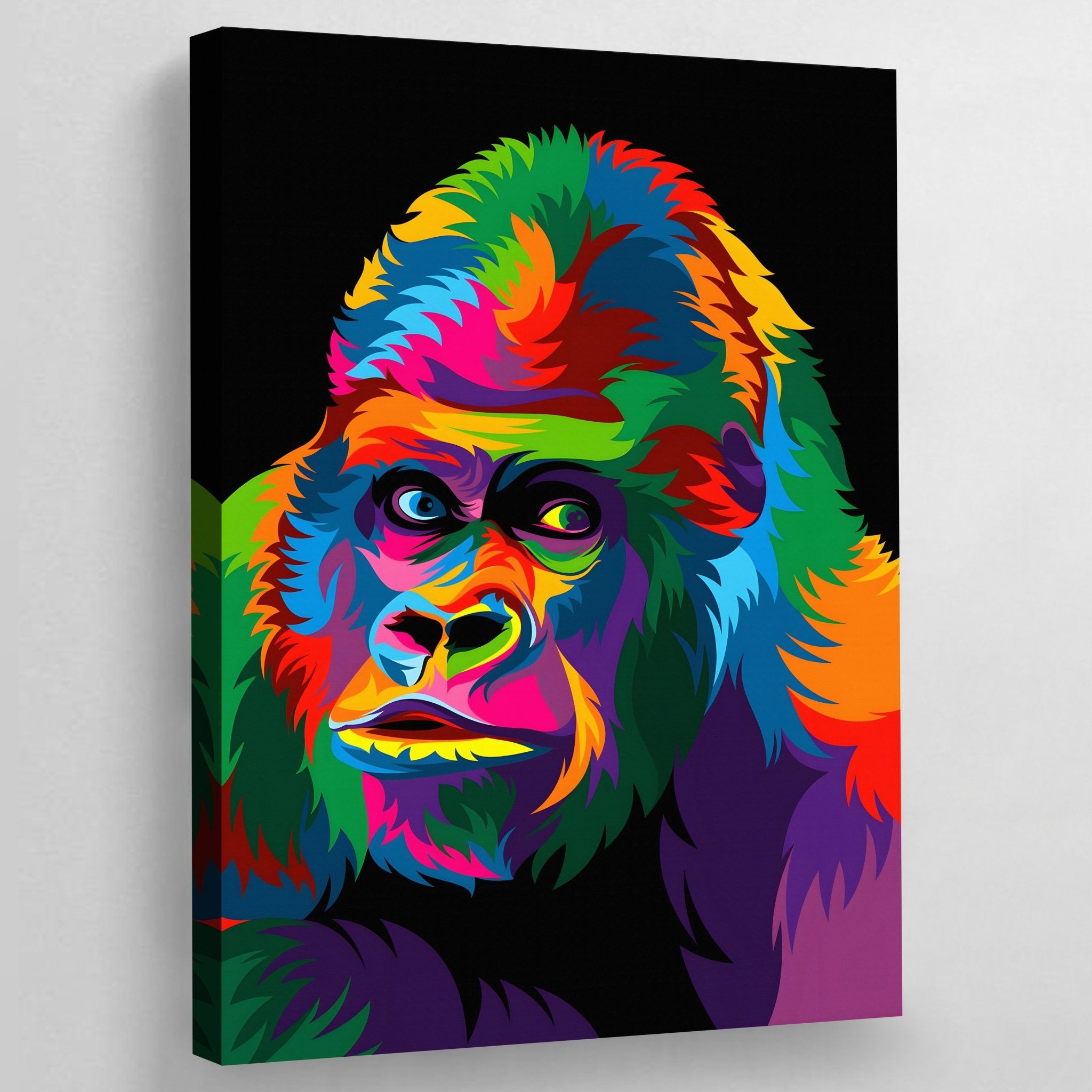This image features a vibrant, multicolored, pop art style print of a gorilla, displayed at an angle on a raised black canvas. The focal point of the artwork is the gorilla's head, which is prominently detailed with an array of vivid colors. The gorilla’s fur showcases a spectrum of colors including purples, pinks, yellows, greens, blues, reds, and oranges. Its eyes are distinctly different colors, one blue and one green, adding to the striking nature of the piece. The print features the head and shoulders of the gorilla, with even the fur's intricate details wrapping around the sides of the canvas, creating a fully immersive effect. The canvas itself is mounted on a white wall, suggesting a gallery or modern exhibition setting.